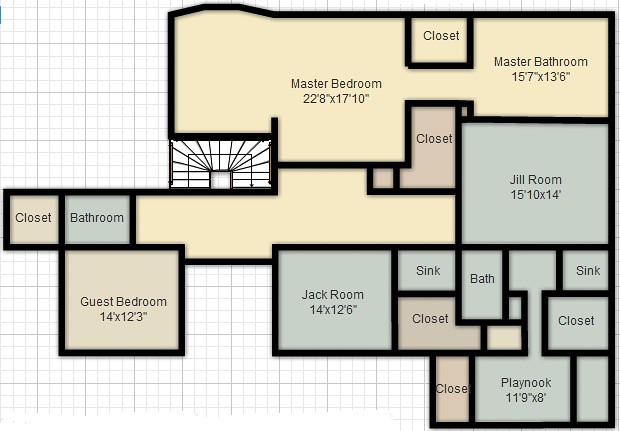This image depicts a detailed floor plan of a house overlaid on graphing paper visible in the upper left corner. The floor plan sketch employs a pale pink and pale blue color scheme, with room outlines highlighted in bold black lines for clarity. 

At the top of the layout is the master bedroom, which measures 22 feet 8 inches by 17 feet 10 inches. This spacious room leads directly into an adjoining master bathroom, sized at 15 feet by 7 feet and 13 feet by 6 inches. Flanking the hallway adjacent to the master suite are two sizable closets.

Adjacent to the master suite are smaller rooms intended for children, labeled as the “Jack room” and the “Jill room.” These rooms are comparable in size to the master bathroom and each features its own closet. The two children's rooms share a conveniently located bathroom.

Additional features of the floor plan include a cozy play nook and a guest bedroom, rounding out the comprehensive layout designed for both functionality and comfort.